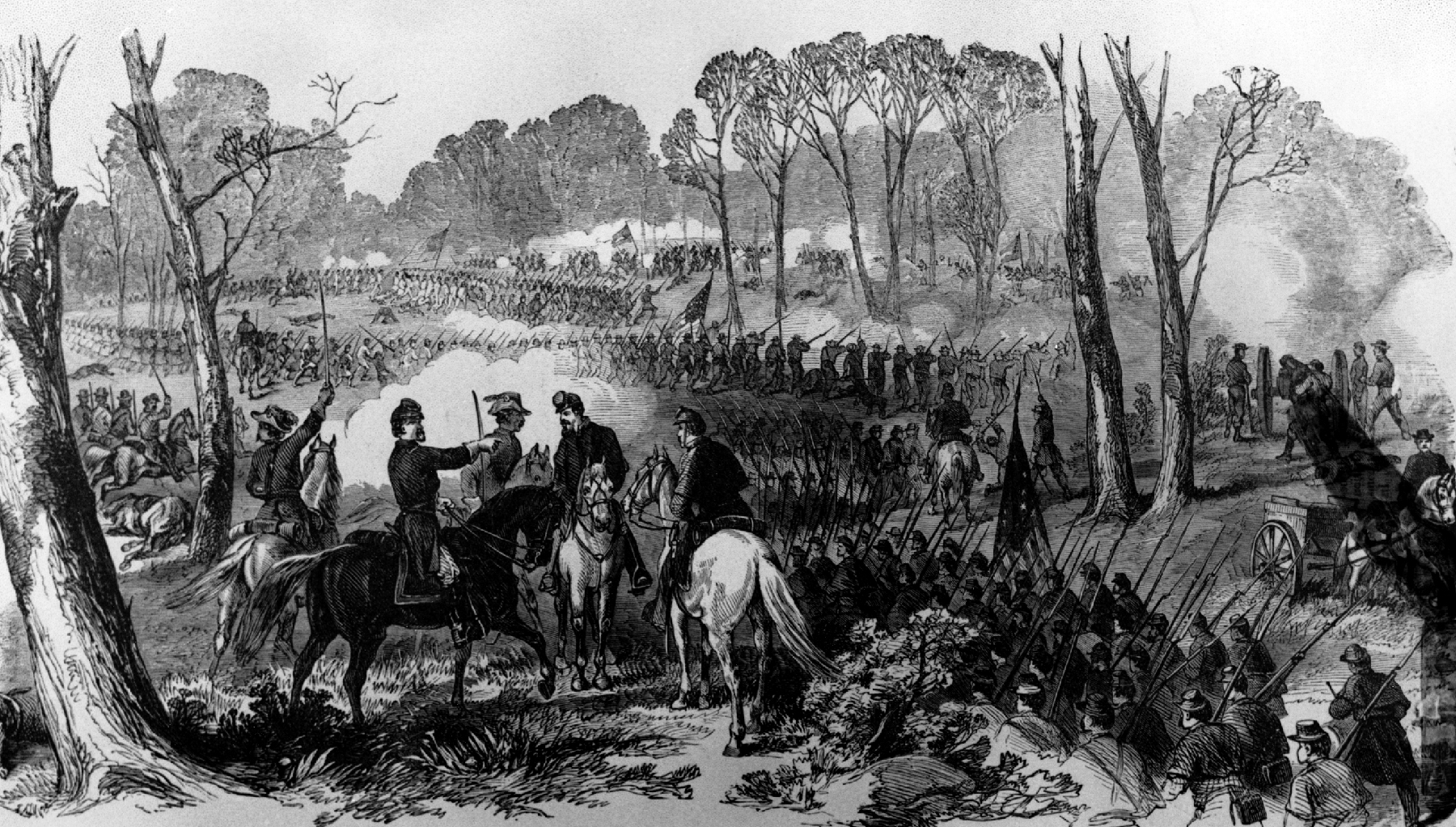The image is a detailed and elaborate black-and-white drawing, evocative of illustrations seen in old school textbooks, potentially depicting a scene from the Civil War. In the foreground, several soldiers are mounted on horses, both black and white, with swords drawn, appearing to be strategizing their next move amidst the ongoing battle. To the right, a large contingent of foot soldiers stands ready, some carrying guns, while others manage a visible cannon. In the background, enemy forces approach, waving flags and brandishing weapons. The scene is set within a clearing surrounded by tall trees, adding a rich texture to the backdrop. Amidst the chaos, soldiers can be seen camping, strategizing, and guarding their positions, creating a vivid portrayal of a historical battlefield scene full of action and tension.